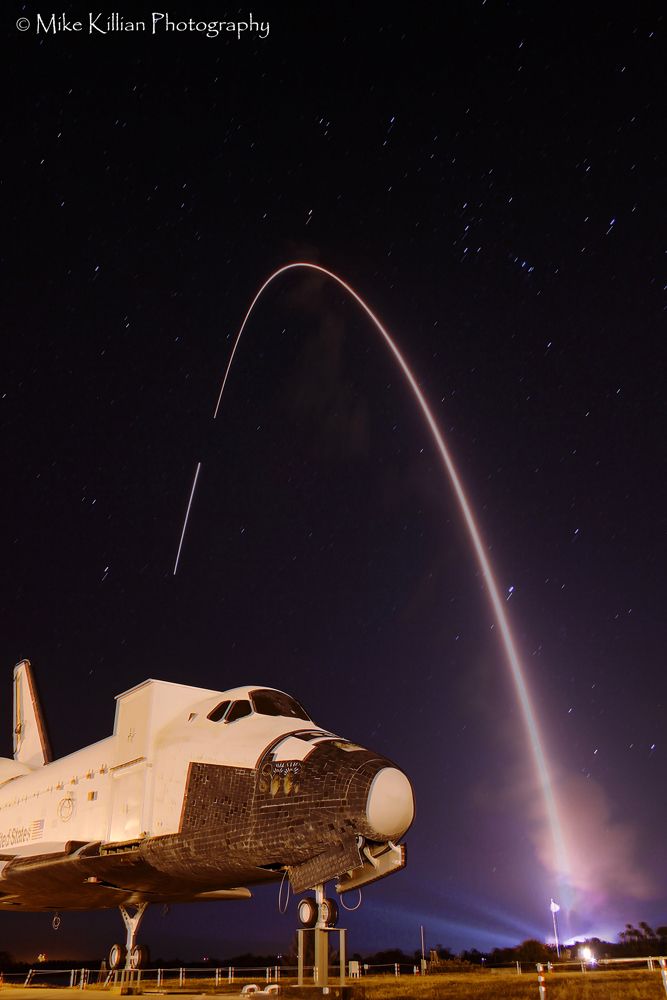The photograph, rectangular in shape with the longer sides stretching horizontally, captures a nighttime outdoor scene dominated by an atmospheric display of an old decommissioned rocket ship. Positioned in the bottom left corner, the rocket ship stands on three large supports. Its body is primarily white, with the nose and underside sheathed in black protective covering, emphasizing its worn, historical nature. The spaceship features a prominent white fin at the back and bears the inscription "United States" alongside a backward-facing American flag in vivid red, white, and blue. Visible through its black-tinted cockpit windows, the rocket's landing gear is deployed, resting on a brownish ground that fades into slight blur near the base, suggesting metal fencing or stands. The night sky enveloping the scene is a blackish purple canvas, punctuated with stars, and traversed by a spectacular streak of light. This light, whitish with purplish hues, originates from the bottom right corner, ascends midway through the sky, curves gracefully, and descends again, creating an ethereal arc. Additional spotlights in the background illuminate the surrounding area, adding to the image's otherworldly ambiance.